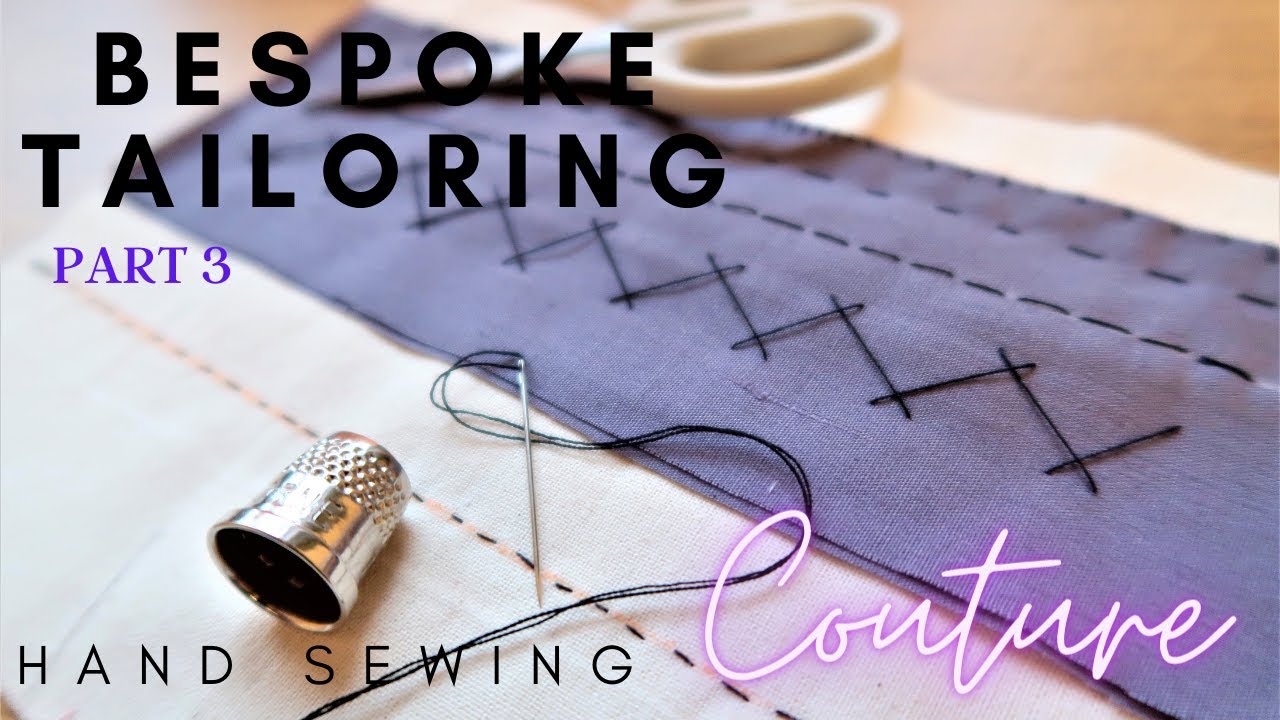The vibrant, professionally composed photograph showcases a meticulously staged assortment of sewing tools and materials on a likely brown table. Central to the image is a strip of blue fabric, adorned with various hand-sewn stitches, emphasizing the art of hand sewing. Piercing through the fabric is a needle threaded with black thread, looping gracefully, while a shiny silver thimble, used to protect fingers from needle pricks, sits nearby. A pair of scissors with distinctive white handles adds to the array of tools. Text overlays the image prominently: at the top, bold white letters read "Bespoke Tailoring Part 3 Hand Sewing," suggesting this image is part of a how-to guide series. Adding a touch of flair, the word "Couture" is illuminated in a purple and white Vegas-style light script at the bottom right, reinforcing the theme of personalized, high-quality garment creation.